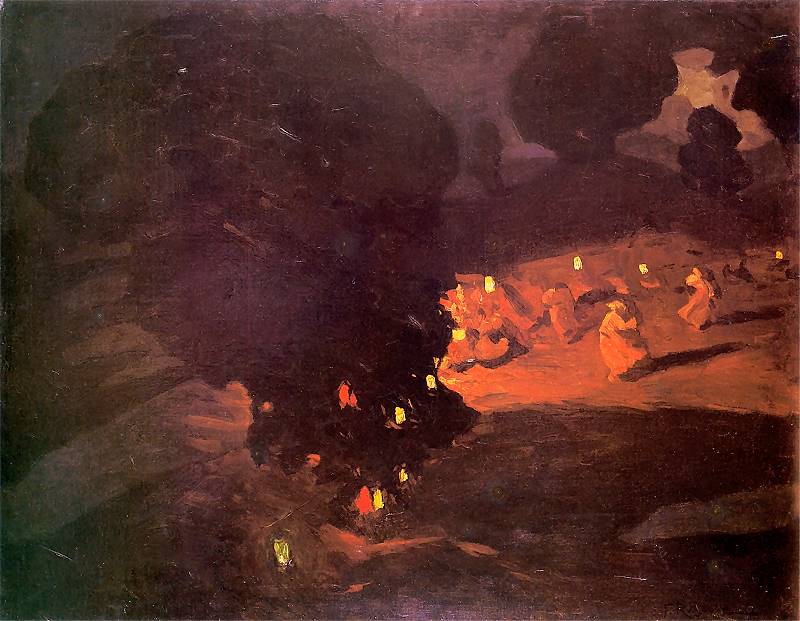This painting depicts a sinister nighttime scene dominated by dark, reddish-black hues, evoking a sense of foreboding. Central to the painting is a large bonfire with intense, billowing black smoke rising prominently toward the left, illuminating the surrounding area with its fiery glow. Around this bonfire, a group of roughly ten hooded figures, possibly evoking sinister historical connotations, are gathered. Most hold torches aloft, casting flickering yellow and orange light that clashes starkly against the overall dark maroon, red, and black tones of the painting. The figures are robed, with one notable figure in a white robe standing behind the bonfire, adding to the eerie atmosphere. To the right, bursts of deep orange flames protrude, emphasizing the fire's intensity. The treeline in the background is depicted as mere black shadows, with one prominent tree crowning a small hill that slopes down to the path where the robed figures walk. Lone lanterns dot the scene, their faint light barely piercing the surrounding darkness. The sky above is marked with shadowing effects, possibly indicative of smoke spreading outwards, adding to the painting's overall dark and mysterious ambiance.